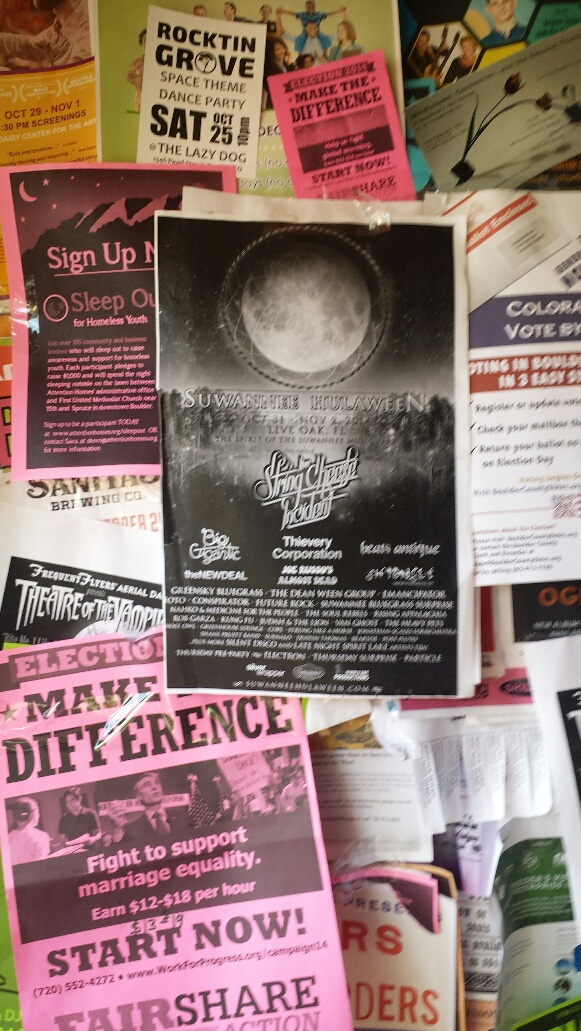The image depicts a vertical bulletin board filled with various overlapping promotional posters, largely in an outdoor or indoor setting. Dominating the center of the board is a prominent black and white flyer advertising Suwannee Hulaween with a large moon and a dreamcatcher at the top, followed by the name of the event in bold white letters. Below this central flyer, the band name, The String Cheese Incident, appears in cursive print alongside sponsors' names. Surrounding this main flyer, numerous 8.5x11 event posters and smaller business cards add to the collage, including a poster for a Rockton Grove Space-Themed Dance Party on October 25th at the Lazy Dog and multiple signs promoting an Election with a call to action supporting marriage equality with wages ranging from $12-$18 an hour. A bright yellow poster announcing October 29th and November 1st PM Screenings lies towards the upper left, while a green flyer featuring a family photo peeks from behind. The layers of diverse colored posters—pink, purple, gray, green, red, orange, yellow, blue, and maroon—collectively create a visually chaotic yet intriguing collage, making some details hard to discern.